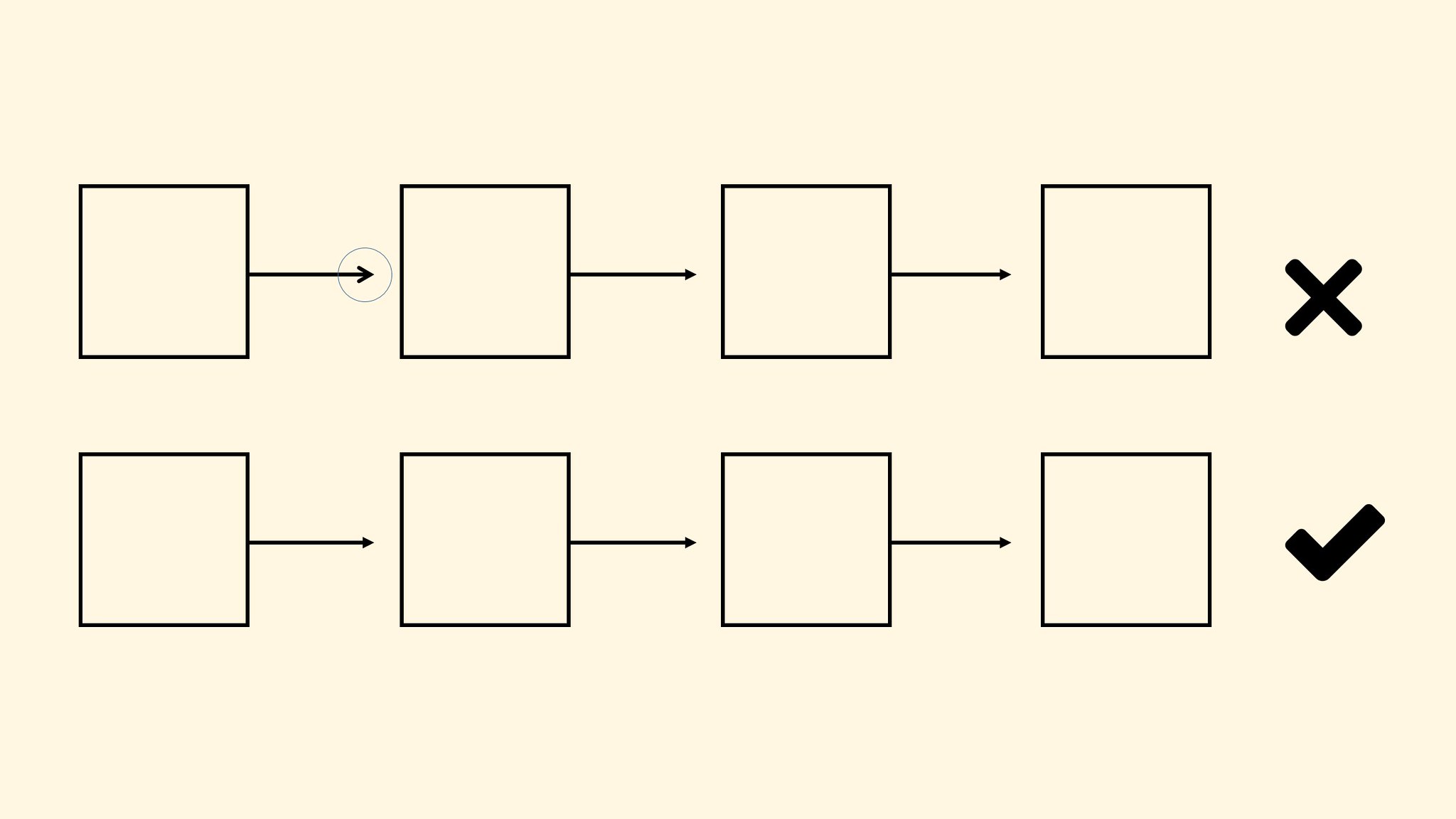This is a beige and black schematic drawing. On the top left, there is an outlined black box, followed by a black arrow pointing to the right. A light gray circle partially encircles the top part of the arrow. To the right of this arrow is another outlined black box, matching the first one in color with a beige interior. Another black arrow emerges from this second box, extending into an open space before leading to a third outlined black box. Continuing rightwards, another black arrow guides the eye through an open space to a fourth black box, all of which share the same beige interior. To the right of this final box in the sequence, there is a thick black X.

In the lower section of the drawing, a similar sequence of outlined black boxes and arrows unfolds. A black box is present on the left, followed by a right-pointing black arrow that extends into an open area before reaching a second black box. Another right-pointing arrow comes from this box, leading to a third outlined black box through yet another open space. This pattern continues with a fourth black box and another arrow pointing to the right, which also ends in an open space before the fifth and final black box appears to the right. Adjacent to this last box is a thick black check mark, identical in darkness and width to the X seen in the upper section.